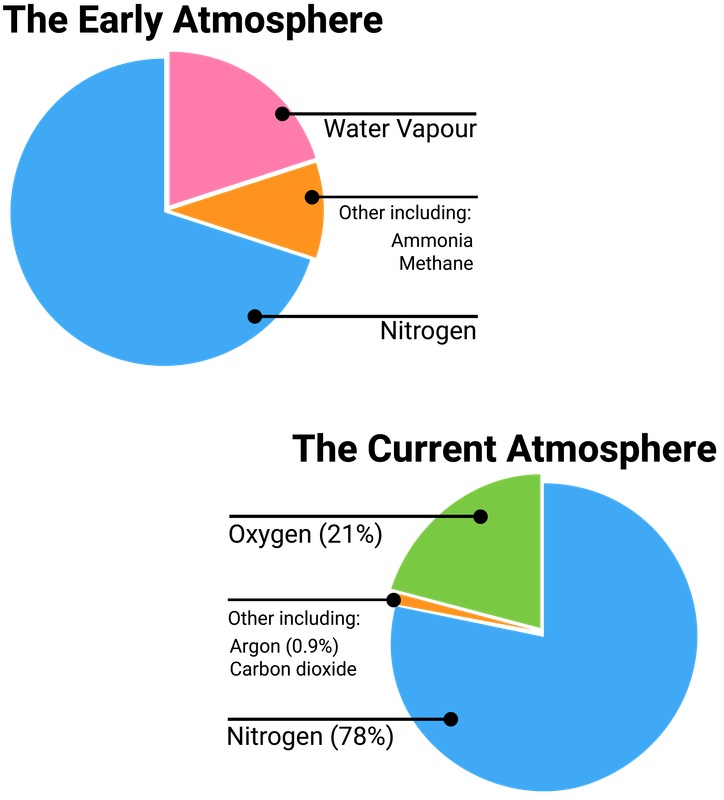The image features two detailed pie charts illustrating the composition of the Earth's atmosphere across two different eras. 

The top left pie chart, titled "The Early Atmosphere," is divided into three distinct sections. A pink segment, labeled "Water Vapor," occupies approximately one-sixth of the chart. Below it, an orange section, labeled "Other," includes gases like ammonia and methane and covers around 10% of the pie. The remaining, dominant blue section represents "Nitrogen," which makes up about 65% of this early atmospheric composition.

The lower right pie chart, titled "The Current Atmosphere," depicts the modern composition. The largest section in blue, labeled "Nitrogen," constitutes 78% of the chart. A green segment, labeled "Oxygen," covers 21%. The smallest portion, an orange sector labeled "Other," includes gases such as argon and carbon dioxide, representing 0.9% of the current atmosphere. 

Both charts have a thin white outline around each slice, with black text labels pointing to the relevant sections. Lines extend from these labels, intersecting with circles that touch each section of the pie charts, visually connecting the text to the corresponding atmospheric components.